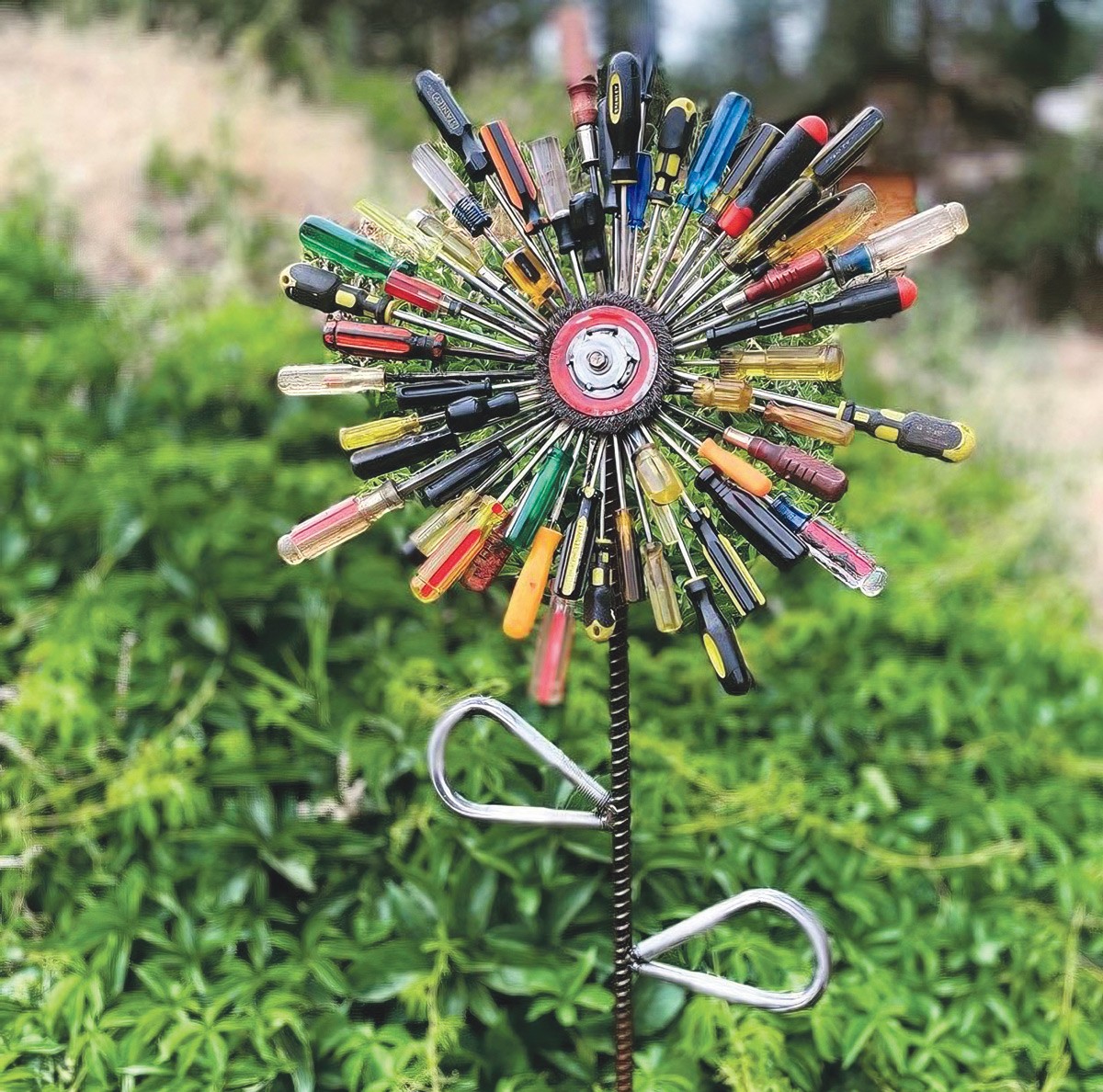This photograph captures a unique piece of yard art crafted from ordinary hand tools and metal. Situated outdoors against a backdrop of blurred tree trunks and a mix of green and wheat-colored grass, the central artwork features a flower constructed from an array of multicolored screwdrivers. These screwdrivers, with handles in hues of black, yellow, red, yellow and black, clear, green, and blue, radiate outwards from a central grinding wheel. The flower's stem is a piece of dark-colored rebar, with teardrop-shaped silver metal pieces on either side, mimicking leaves, creating a striking and intricate sculpture.